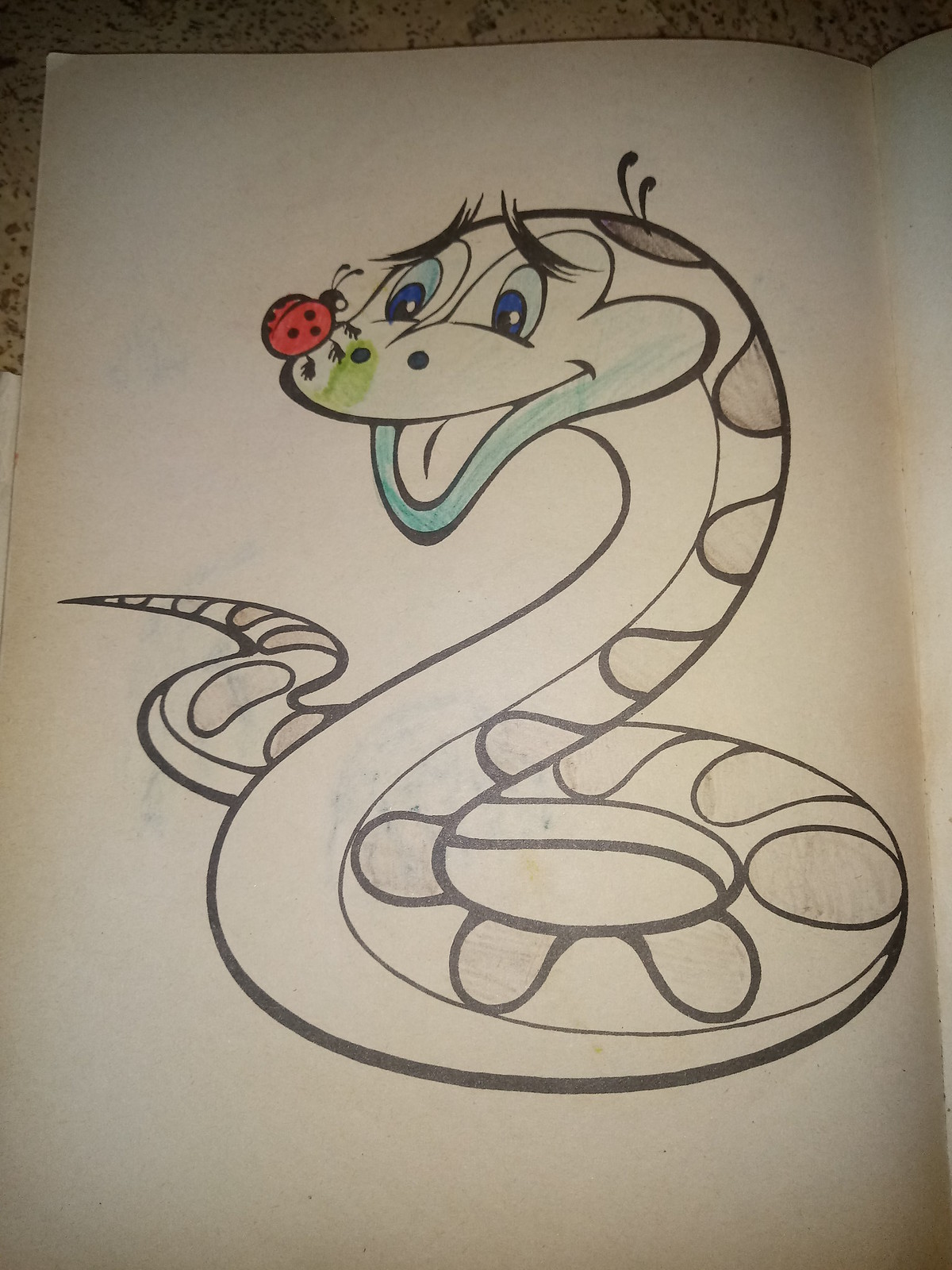The image captures a page from a children's coloring book set on a beige, granite-like countertop. The primary subjects on the white paper are a cheerful snake and a ladybug. The snake, with a white underbelly, coils and curves in a friendly posture, smiling warmly at the ladybug perched on its nose. The snake's eyes are a mix of light and dark blue, with a light blue mouth and a human-like tongue poking out. Uniquely, the snake has two small antennae on its head. The ladybug is meticulously colored in red, with a black head, antennae, feet, and three black spots on its back. The snake's head includes some green coloring on the nose. Some of the snake's body has gray circles filled in, suggesting the drawing is partially complete. The overall scene evokes a playful and whimsical interaction between the two creatures.